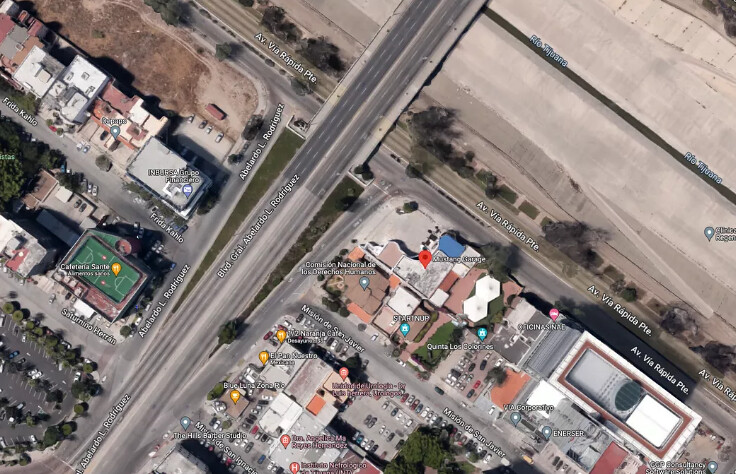An aerial photograph, likely captured using a drone, showcases a sprawling town from a high vantage point. In the center of the image, a three-lane highway, labeled "Boulevard Abelardo L. Rodriguez," cuts diagonally across the landscape, distinguishing itself with its concrete structure. Flanking this thoroughfare, lush green trees add a touch of natural beauty and contrast to the man-made surroundings.

To the left side of the highway, the tops of various buildings are clearly visible, varying in architectural styles and sizes. One prominent feature is a rectangular sports area, predominantly green, that could either be a tennis court or a soccer field. A distinct yellow object, perhaps equipment or decoration, stands out on this field, drawing immediate attention.

Dominating the right side of the photograph is a significant waterway known as "Rio Tijuana," which winds its way through the town, contributing to the area's geography and ecosystem. The detailed landscape, with its blend of urban and natural elements, provides a comprehensive view of the town's layout and key points of interest.

This descriptive caption encapsulates the essence of the aerial view, highlighting important features and landmarks while providing a clear, detailed narrative of the scene.